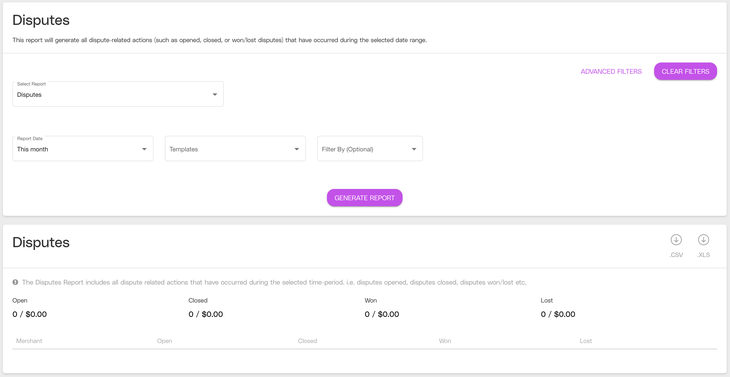The webpage features a predominantly white background, with a black text heading labeled "Disputes" in the top left corner. Below the header, there's a concise description in small black text stating: "This report will generate all dispute-related actions such as opened, closed, or won/lost disputes that have occurred during the selected date range." 

A horizontal line spans the width of the page, dividing the header from the interactive content below. The section that follows contains various dropdown boxes for filtering disputes by criteria such as "This Month," "Templates," and an optional "Filter By." In the upper right corner of this section, a purple button labeled "Advanced Filters" is visible, accompanied by a similarly colored rectangular button that appears to be selected and reads "Clear Filters."

At the bottom of the filter section, another purple rectangular button labeled "Generate Report" is prominently displayed.

The next section, also headed "Disputes" in black text, offers file download options on the right side. Two circle icons with downward arrows indicate options to download the report in either CSV or XLS formats. Below this, a line of lighter gray text, smaller in size, reiterates: "The disputes report includes all dispute-related actions that have occurred during the selected time period, i.e., disputes opened, disputes closed, disputes won/lost, etc."

Finally, a summary section features counters indicating the status of disputes with corresponding monetary values. The statuses include: "Open: 0 / $0," "Closed: 0 / $0," "Won: 0 / $0," and "Lost: 0 / $0."